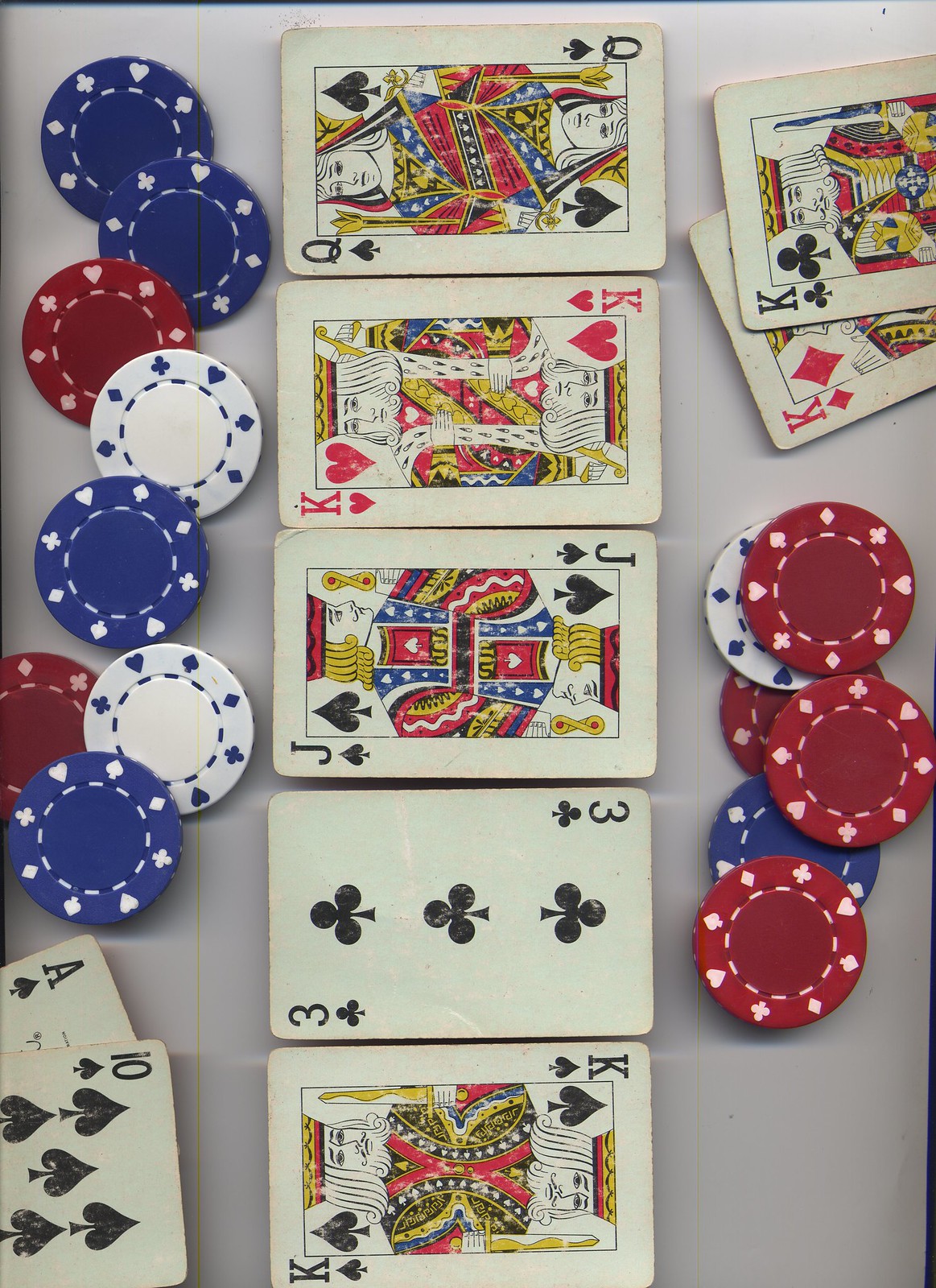This vibrant color photograph captures an intriguing poker scene viewed from a slightly unconventional angle. At the heart of the image, a row of playing cards runs horizontally across the frame, featuring an assortment of mostly face cards: two kings, a jack, a queen, and a three of clubs. These cards are oriented vertically, creating a striking central column.

Flanking this central column is a lively arrangement of poker chips and additional playing cards. On the right side, the exposed hand shows a king of diamonds and a king of clubs, alongside a cluster of four red chips, one blue chip, and a white chip adorned with blue markings. Similarly, the left side displays an array of chips—four blue, two red, and two white—complemented by the ace of spades and the ten of spades lying face up.

The entire setup rests on a pristine white surface, bordered by glimpses of blue along the right and top edges, adding an extra layer of depth and color to the composition. The detailed arrangement and vibrant colors of the cards and chips draw the viewer into the dynamic and suspenseful moment of a poker game.